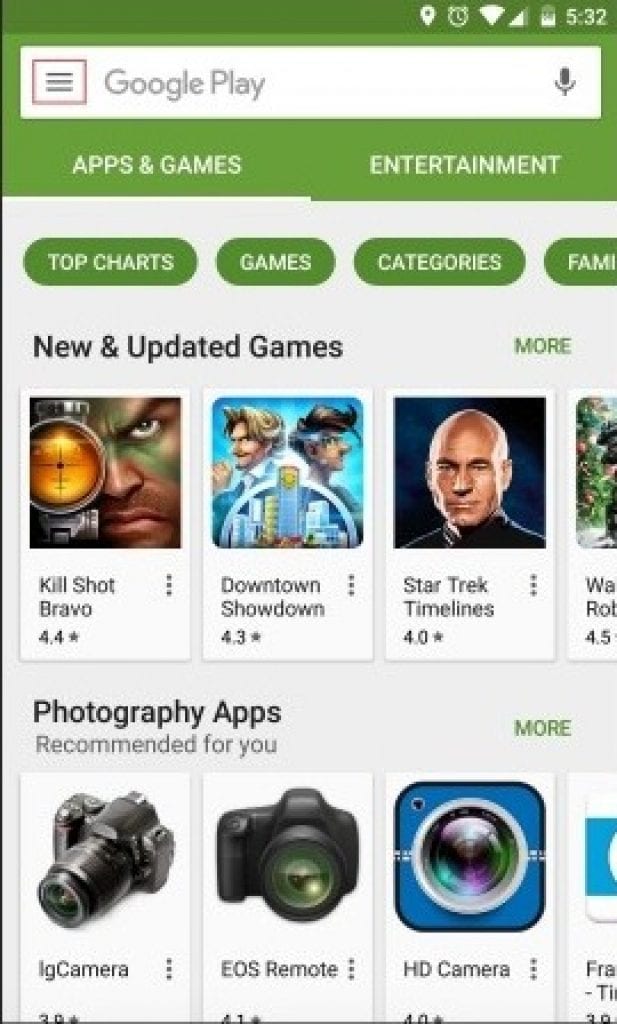This vertical rectangular image is a detailed depiction of an interface likely pertaining to a mobile app store. The top quarter of the image features a light green background. Centered within this green area is a white horizontal rectangle bearing the text "Google Play" in light gray letters. To the left of the "Google Play" text, there is a small reddish-brown outlined box containing three horizontal lines. On the right side, there is a gray microphone icon.

Below this section, still within the light green background, are two sets of capitalized text: "APPS & GAMES" on the left and "ENTERTAINMENT" on the right.

The remaining portion of the image expands on a white background. Starting from the top, there are four horizontal green ovals with white, capitalized text inside them. These ovals are sequentially labeled "TOP CHARTS," "GAMES," "CATEGORIES," and "FAMILY," though the last word is partially cut off by the edge of the image. 

Under these ovals, "NEW & UPDATED GAMES" is boldly written in black, with a green, capitalized "MORE" to its right. Beneath this heading, there is a display of games, showcasing vertical rectangular images with text descriptions under each. 

1. The first game features an image of a man looking through a telescope and is labeled "Kill Shot Bravo," rated 4.4 stars.
2. The second game has a turquoise background with two men standing back-to-back, labeled "Downtown Showdown," rated 4.3 stars.
3. The third game shows a man against a dark background, labeled "Star Trek Timelines," rated 4.0 stars.
4. The fourth game is partially cut off and unreadable.

Further down, in black text, "PHOTOGRAPHY APPS" is followed by the gray text "RECOMMENDED FOR YOU," with another green "MORE" to the right. This section showcases four camera-related apps, each represented by an image but with their star ratings cut off. The apps are labeled as follows:

1. "IG Camera"
2. "EOS Remote" with only the "R" capitalized
3. "HD Camera" with both "H" and "D" capitalized

Overall, the image meticulously categorizes and displays sections of an app marketplace, highlighting new games and suggested photography apps along with their ratings and icons.